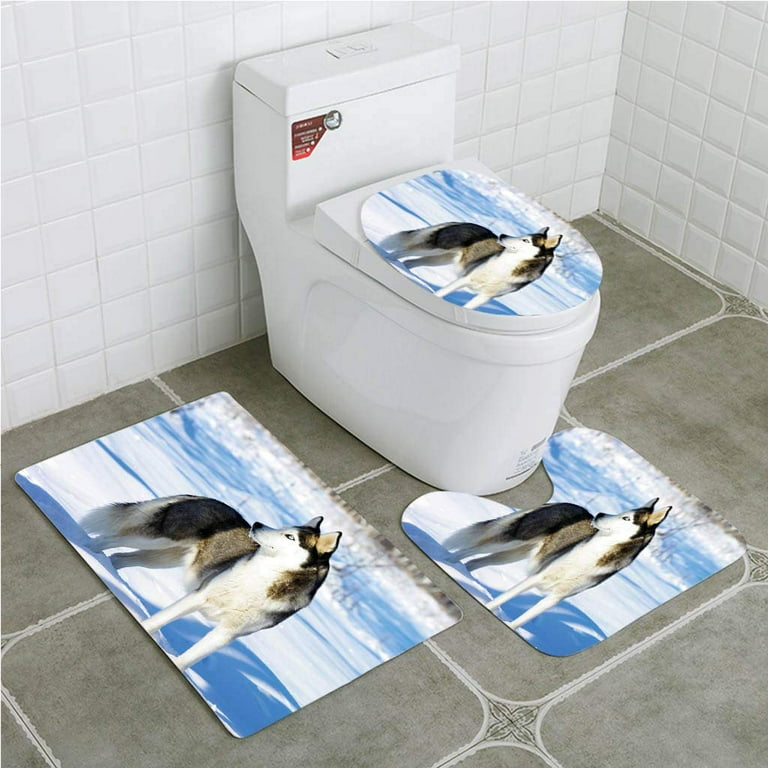The image depicts the inside of a bathroom featuring a modern, white-colored bidet with a closed seat cover. The bidet has a tank that extends to the floor, equipped with a push button and an instructional sticker in red and black for flushing. Surrounding the bidet are three decorative mats, each showcasing a stunning photograph of a husky dog against a snowy, icy background. One mat, rectangular in shape, is placed on the toilet lid; another, with a cutout to fit around the base of the toilet, lies in front; and the third, the largest, is situated to the side of the bidet. The bathroom floor is adorned with large, dark gray ceramic tiles featuring a white square-patterned motif, while the walls are covered with small, white ceramic tiles. The husky dog, beautifully featured on all three mats, has a striking black, gray, and brown coat with a white snout, face, chest, and paws. The dog, standing on what appears to be a partially frozen lake, is looking off to its left, displaying an alert expression with its pointed ears upright. The detailed and cohesive decor highlights the intricate and harmonious interplay between the bathroom's modern fixtures and the artistic flair of the husky-themed mats.